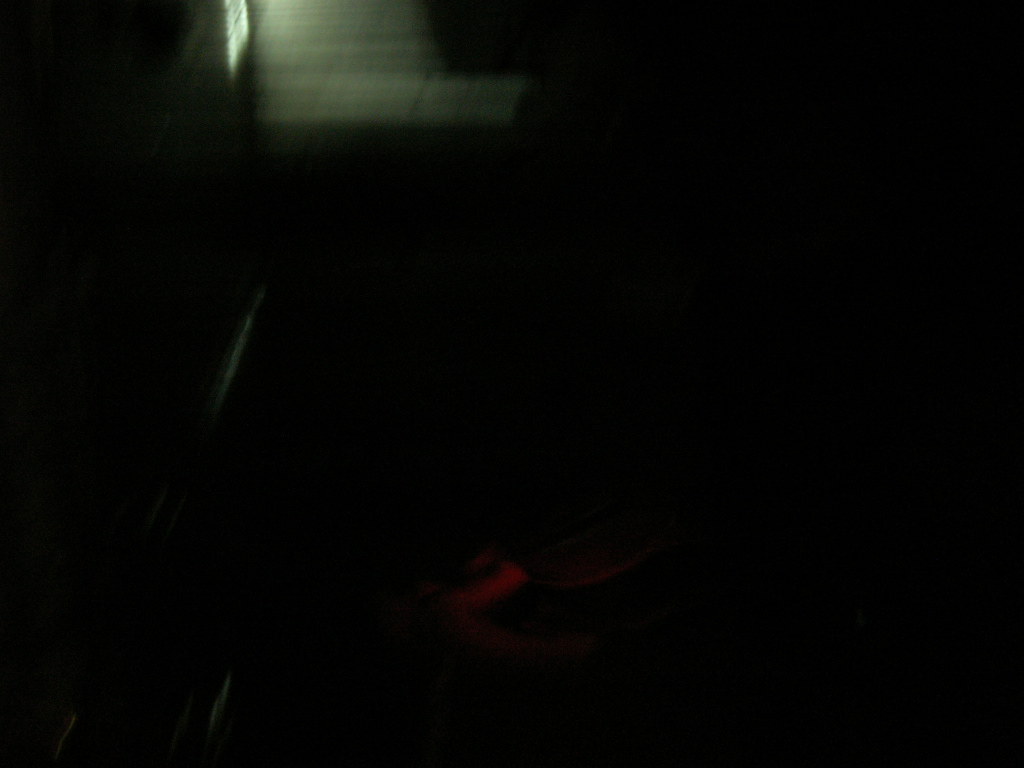This photograph, likely taken outdoors at night, is predominantly enveloped in darkness, with approximately 94% of the image composed of blackness, rendering it difficult to discern shapes or depth. In the top left corner, there's a small, illuminated rectangular area emitting a greenish light, possibly from a window or grate, which casts a soft glow onto the surrounding area. Directly below this rectangle, several small streaks of similar greenish light can be seen, while towards the center bottom of the image, there are wider streaks of red light, giving the impression of reflections or faint illuminations in the obscurity.